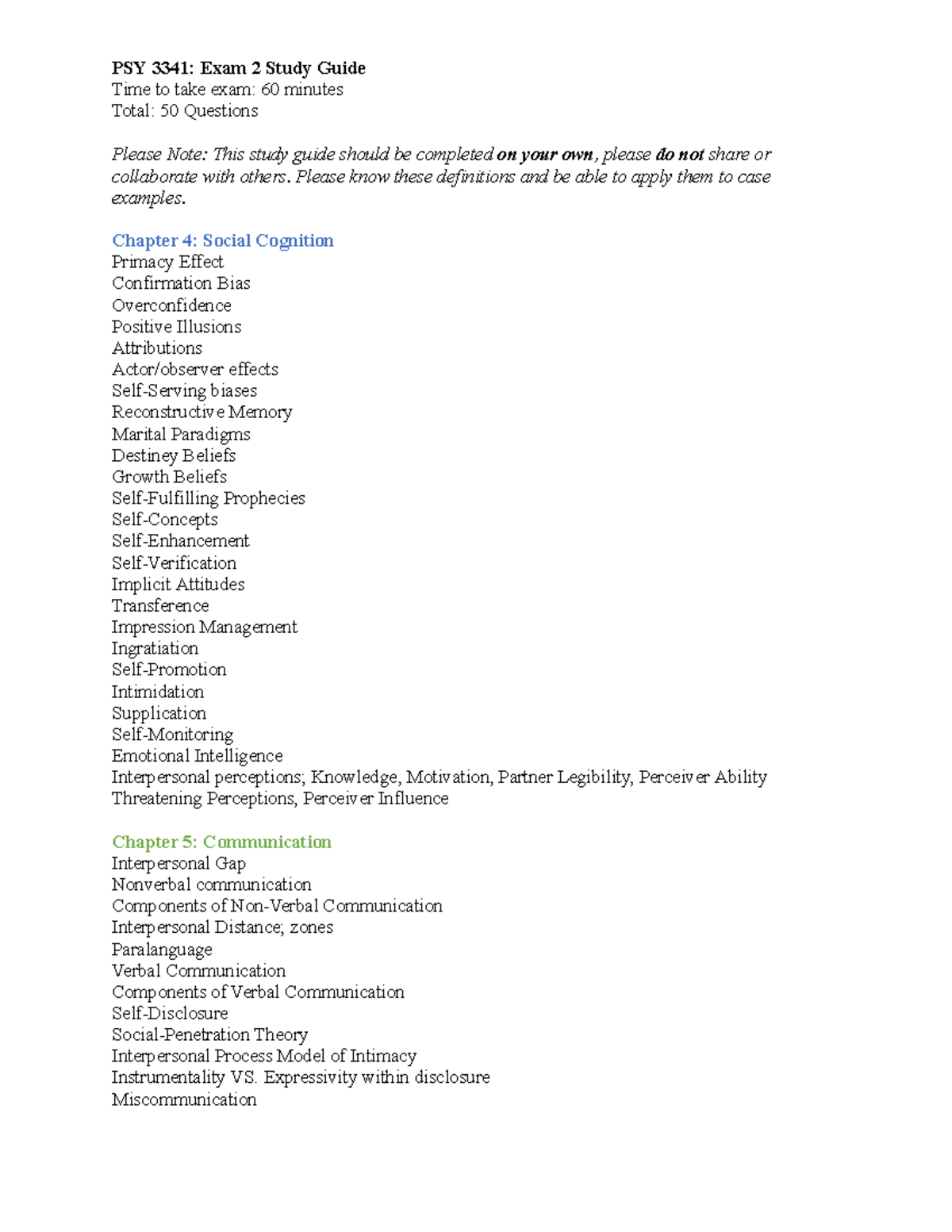This is a detailed photograph of a white web page designated as a study guide for an exam in PSY3341. 

At the top of the page, prominently displayed in bold black text, is the title: "PSY3341 - Exam 2 Study Guide." Beneath it, regular black text provides additional details: "Time to take exam: 60 minutes; Total: 50 questions." 

Emphasizing the importance of individual effort, italic black text relates the following note: "Please note: This study guide should be completed on your own." This is further reinforced by bolded regular text warning: "Please do not share or collaborate with others. Please know these definitions and be able to apply them to case examples."

The document initiates the content with the heading in blue text, "Chapter 4: Social Cognition." Returning to black text, a list of key terms and concepts under this chapter ensues, formatted in a cascading list:
- Primary Effect
- Confirmation Bias
- Overconfidence
- Positive Illusions
- Attributions
- Actor/Observer Effects
- Self-Serving Biases
- Reconstructive Memory
- Marital Paradigms
- Destiny Beliefs
- Growth Beliefs
- Self-Fulfilling Prophecies
- Self-Concept
- Self-Enhancements
- Self-Verification
- Implicit Attitudes
- Transference
- Impression Management
- Integration
- Self-Promotion
- Intimidation
- Supplication
- Self-Monitoring
- Emotional Intelligence
- Interpersonal Perceptions

Following a semicolon, the list continues with:
- Knowledge
- Motivation
- Partner Legibility
- Perceiver Ability
- Threatening Perceptions
- Perceiver Influence

Transitioning to the next section, the text appears in green, stating "Chapter 5: Communication." The discussion resumes in black text with another cascading list detailing key concepts in communication:
- Interpersonal Gap
- Nonverbal Communication
- Components of Nonverbal Communication
- Interpersonal Distance Zones
- Paralanguage
- Verbal Communication
- Components of Verbal Communication
- Self-Disclosure
- Social Penetration Theory
- Interpersonal Process Model of Intimacy
- Instruction Ability versus Expressivity
- Width and Disclosure
- Miscommunication

This comprehensive visual captures important study topics for PSY3341's Exam 2, providing a structured guide to assist students in their preparation.